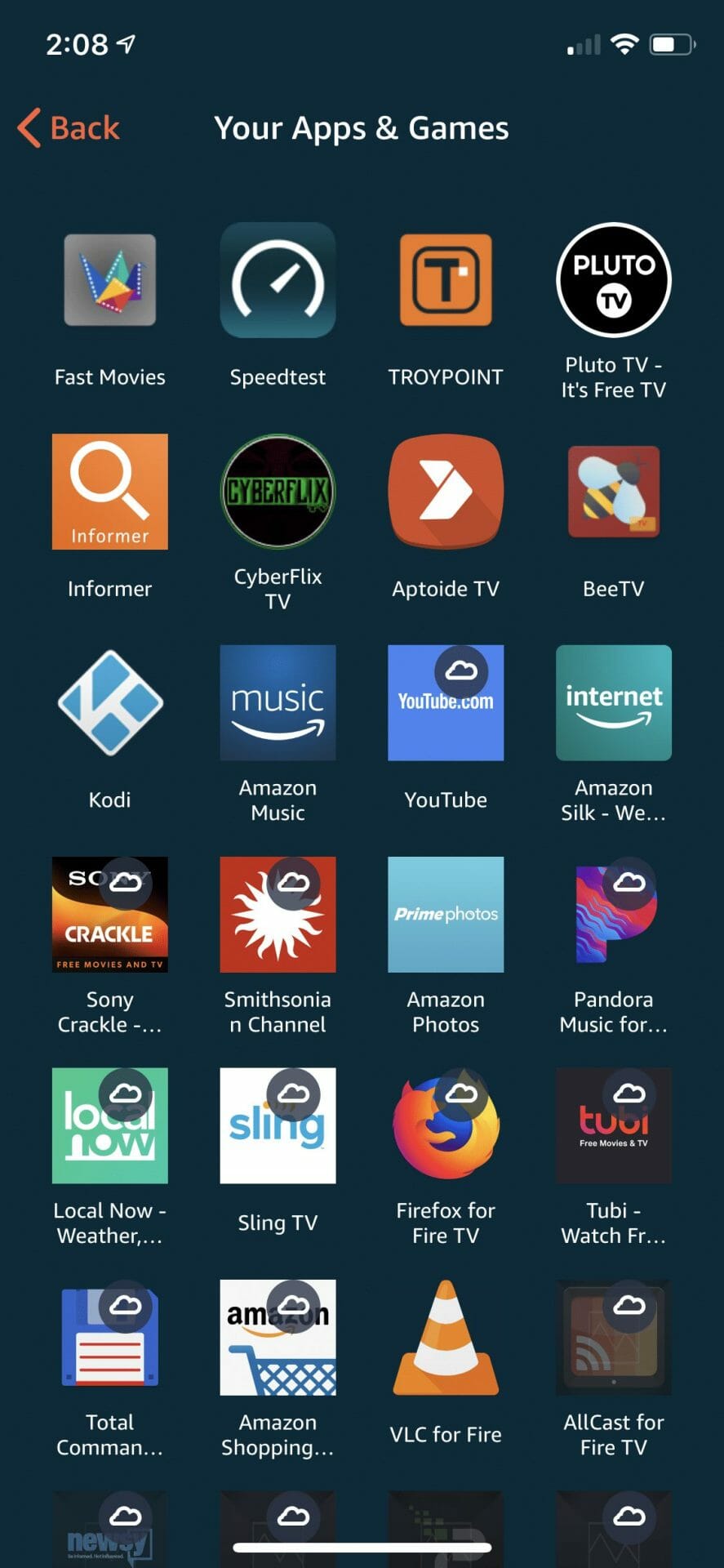This image is a screenshot from a mobile device, displayed in portrait orientation with proportions typical of a smartphone screen. The image has a dark blue background, and at the top, in white font, it displays the number "208" alongside an upward-pointing navigation arrow, which directs towards the right. Adjacent to these elements on the right are a network connection icon with one out of four bars filled, a fully filled Wi-Fi meter, and a horizontal battery indicator showing a white bar more than halfway full.

Below this status bar, there is an orange left-pointing arrow accompanied by the word "Back" in orange text, followed by the label "Your Apps & Games" in white. The main portion of the screen is occupied by a grid layout featuring four columns and approximately six rows of app icons. Each app icon has its respective name displayed beneath it in white text.

The apps listed in this grid are as follows:
- FastMovie
- SpeedTest
- TroyPoint
- Pluto TV
- Informer
- Cybex Films
- Aptitude TV
- BTV
- Kodi
- Amazon Music
- YouTube
- Amazon
- Sony
- Smithsonian Channel
- Amazon Photos
- Pandora Music
- LocalNow
- Sling TV
- Firefox TV
- TubiWatch
- Total Command
- Amazon Shopping
- VLC for free
- Allcast Fire TV

All the app names are accompanied by their icons, which are displayed directly above the textual descriptions.